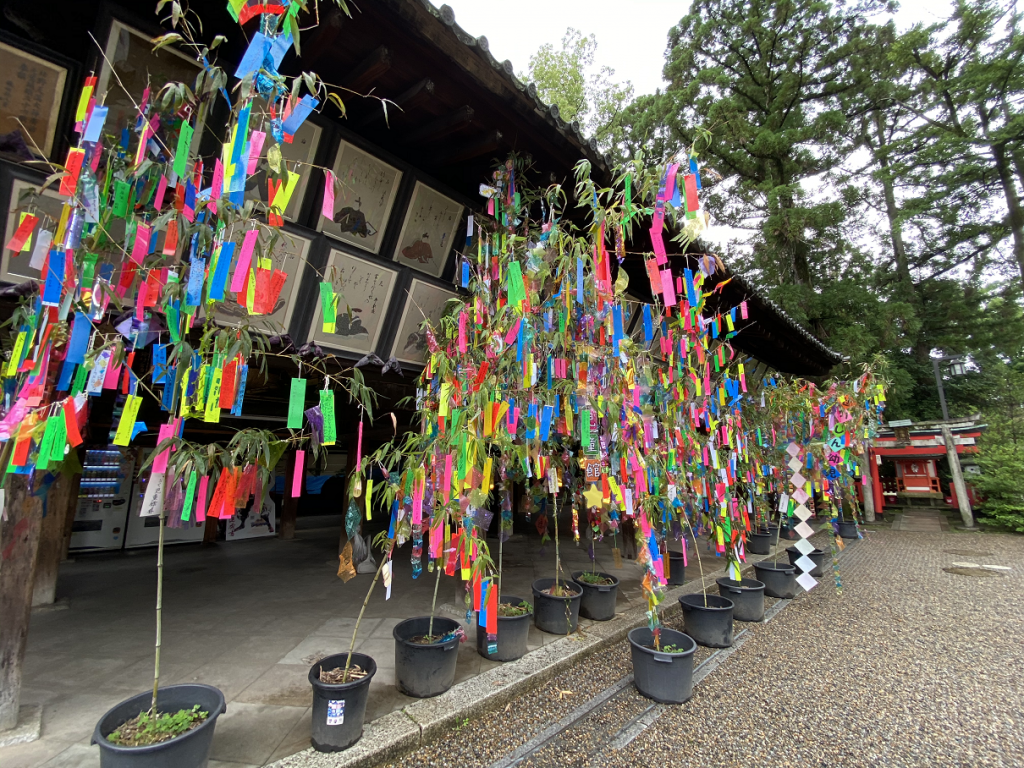This scene captures a bustling display outside what appears to be a shop or possibly a temple on a stone-paved street lined with greenery. Dominating the foreground are two rows of potted sapling trees, likely bamboo, set in black buckets positioned both along the curb and onto the street. Each tree is adorned with vibrant, multi-colored ribbons or paper strips in hues of blue, pink, purple, green, and yellow. These potted plants form a dense barrier that partially obscures the view beyond.

To the left, a building with a traditional Japanese roof features an array of artwork and possibly vending machines beneath its awning, positioned in a two-tiered arrangement. The artwork includes images resembling Asian samurai characters, though they are somewhat distant and not easily discernible. These features contribute to the ambiance, suggesting the locale might be in Japan.

In the background, interspersed among green trees, a striking red torii gate or archway stands prominently, adding a vibrant splash of color and hinting at a cultural or religious significance to the setting. The combined elements evoke a rich, detailed scene indicative of an outdoor market or a cultural display possibly celebrating a festival or significant event.